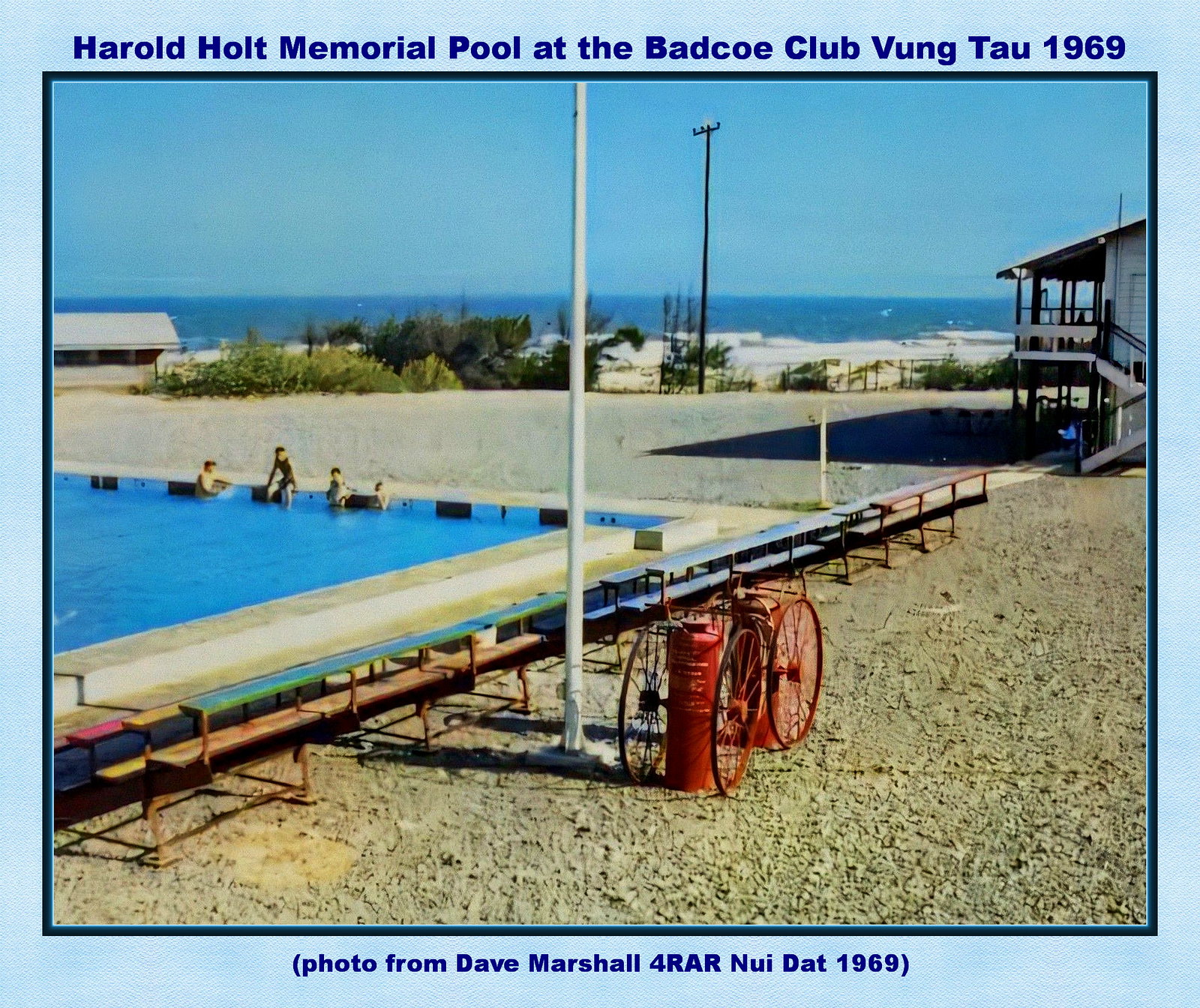The image, styled almost like a poster, is framed in a black frame with a light blue border surrounding it. At the top, in dark blue lettering, it reads "Harold Holt Memorial Pool at the Badco Club, Vung Tau 1969," while the bottom center caption states, "photo from Dave Marshall for RAR Nui Dat 1969."

At the heart of the picture, under a clear, cloudless blue sky, stretches a scenic coastline with the ocean in the background. Closer to the foreground on the left side, a corner of a bright blue swimming pool is visible, where four children lounge, with one sitting at the pool's edge. Surrounding the pool are rows of benches.

In the middle center of the image stands a white pole, likely a flagpole, and to the middle right, two red bicycles are parked next to a bicycle stand. The sandy terrain is dotted with small green bushes, and the landscape features a partial view of a white building with stairs and an awning in the upper right.